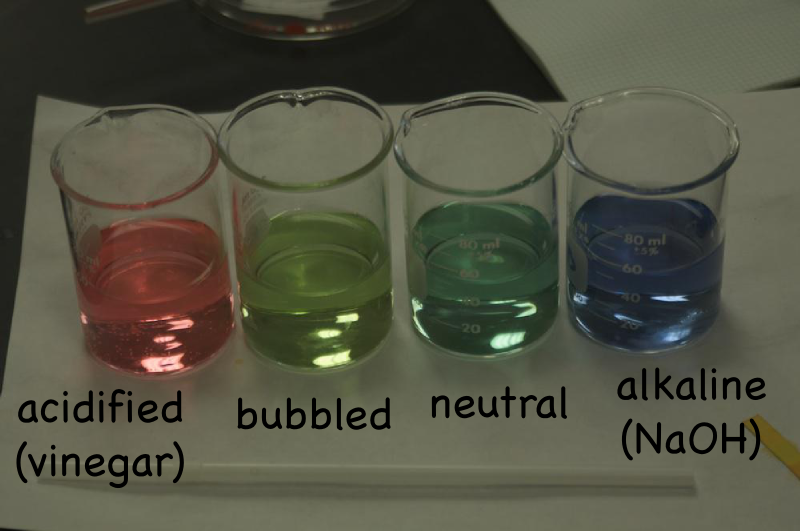In this landscape-oriented color photograph, four clear glass beakers are arranged side by side on a white paper surface, each filled with a distinct colored liquid. From left to right, the liquids are pink, lime green, teal, and blue. Measuring lines on each beaker show volumes ranging from 20 ml to 80 ml. Printed in black text, the labels in front of the beakers describe the contents respectively as: "acidified vinegar" (pink), "bubbled" (lime green), "neutral" (teal), and "alkaline (NaOH)" (blue). NaOH stands for sodium hydroxide. A white tube or straw lies horizontally across the front of the beakers, and in the background, additional white papers and a partially visible black area with a round container edge can be seen. This detailed, representational photograph combines realistic imagery with textual elements to provide a clear and informative depiction of the beakers and their contents.